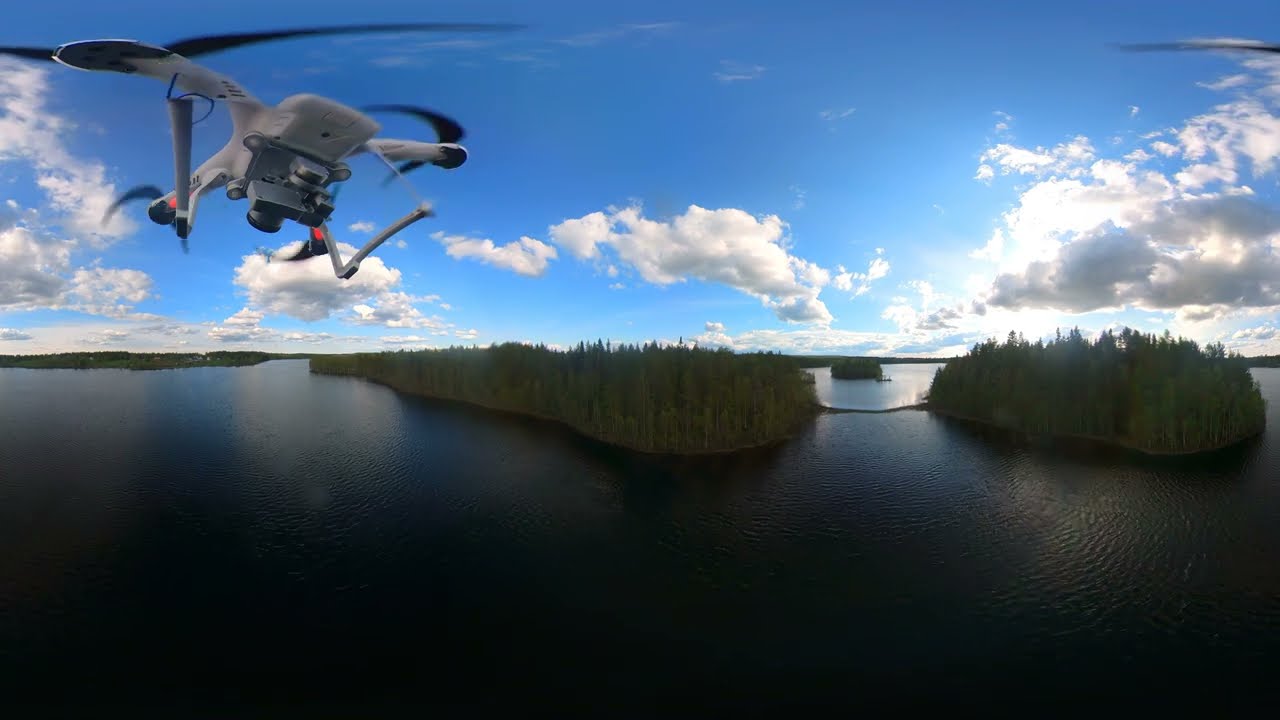This high-angle aerial photograph, likely captured by another drone, showcases a tranquil natural landscape featuring a large lake or swampy body of water. The bottom half of the image is dominated by the dark blue and greenish-gray hues of the water, interspersed with islands and patches of tall green trees and grass, creating a lush, marshy setting. Centrally positioned within the lake is a prominent island densely populated with trees, flanked by another smaller island on the right and additional tree clusters in the distance to the left. The top half of the image transitions into a partly cloudy sky, with a gradient from light to dark blue as it meets the horizon line. Puffy white clouds add to the serene atmosphere, with sunlight peeking through on the right side. Notably, a second drone flies in the top left corner of the image, characterized by its gray, black, and red components, including distinctive black propeller blades and a small silver camera. The overall composition captures the essence of a picturesque, untouched natural environment, as seen from a bird’s-eye view.